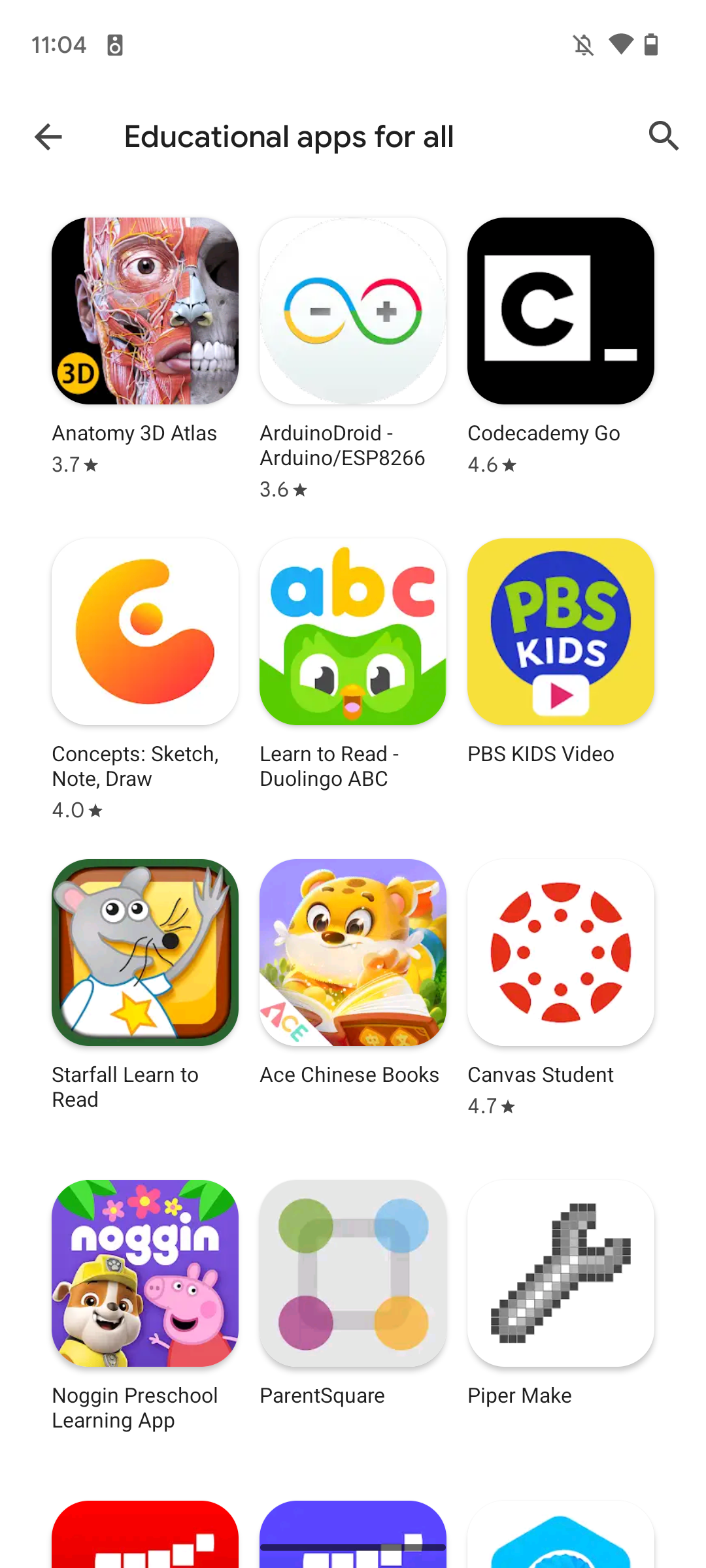This screenshot, captured on a mobile phone, highlights a selection of educational apps available on the device. The top left corner of the image displays the time as 11:04, along with an indistinct picture notification. On the right side, status icons include the sound being off, Wi-Fi connected, and the battery level indicator. The page has a clean, white background with the title "Educational Apps for All" written in bold black letters. To the left of this title, a left-facing arrow serves as a back button, while a magnifying glass icon on the right provides a search function.

The screenshot showcases five rows of educational apps, with three apps neatly arranged per row. The first row includes "Anatomy 3D Atlas," "ArduinoDroid," and "Codecademy Go." The second row repeats "Codecademy Go," followed by "Concepts: Sketch, Note, Draw," and "Learn to Read." The third row displays "Duolingo ABC," "PBS Kids Video," and "Starfall Learn to Read." The fourth row features "Ace Chinese Books," "Canvas Student," and "Noggin Preschool Learning App." The fifth row presents "ParentSquare" and "Piper Make," but the names of the next set of apps in this row are not visible as they are cut off at the bottom of the screenshot.